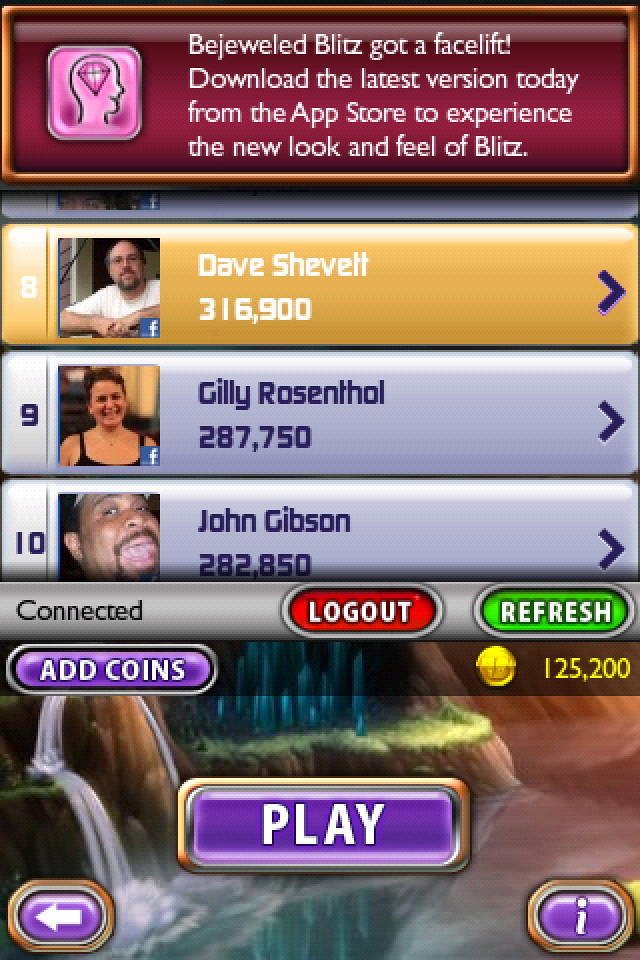The image showcases a vibrant screenshot of the Bejeweled Blitz mobile app, illustrating its newly revamped interface. At the top, against a purple background with a gleaming gold border, white text announces, "Bejeweled Blitz got a facelift. Download the latest version today from the App Store to experience the new look and feel of Blitz." Adjacent to the text, a pink rounded square icon with a diamond illustration inside adds a touch of sparkle.

Below the notification, the screen displays a ranked friends list, each entry containing a profile photo, a name, and a score, accompanied by a blue arrow to the right. Notable scores include Dave Chevette with 316,900 points in eighth place, Jilly Rosendahl with 287,750 points in ninth place, and John Gibson with 282,850 points in tenth place.

Further down, a gray bar labeled "connected" spans the screen, containing a red "log out" button and a green "refresh" button. The interface is enriched by accents of purple: a "play" button centrally located, an "add coins" button in the top left, a "back" button on the bottom left, and an information icon on the bottom right. The total coins, marked as 125,200, are prominently displayed in the top right corner, completing the game's immersive visual update.